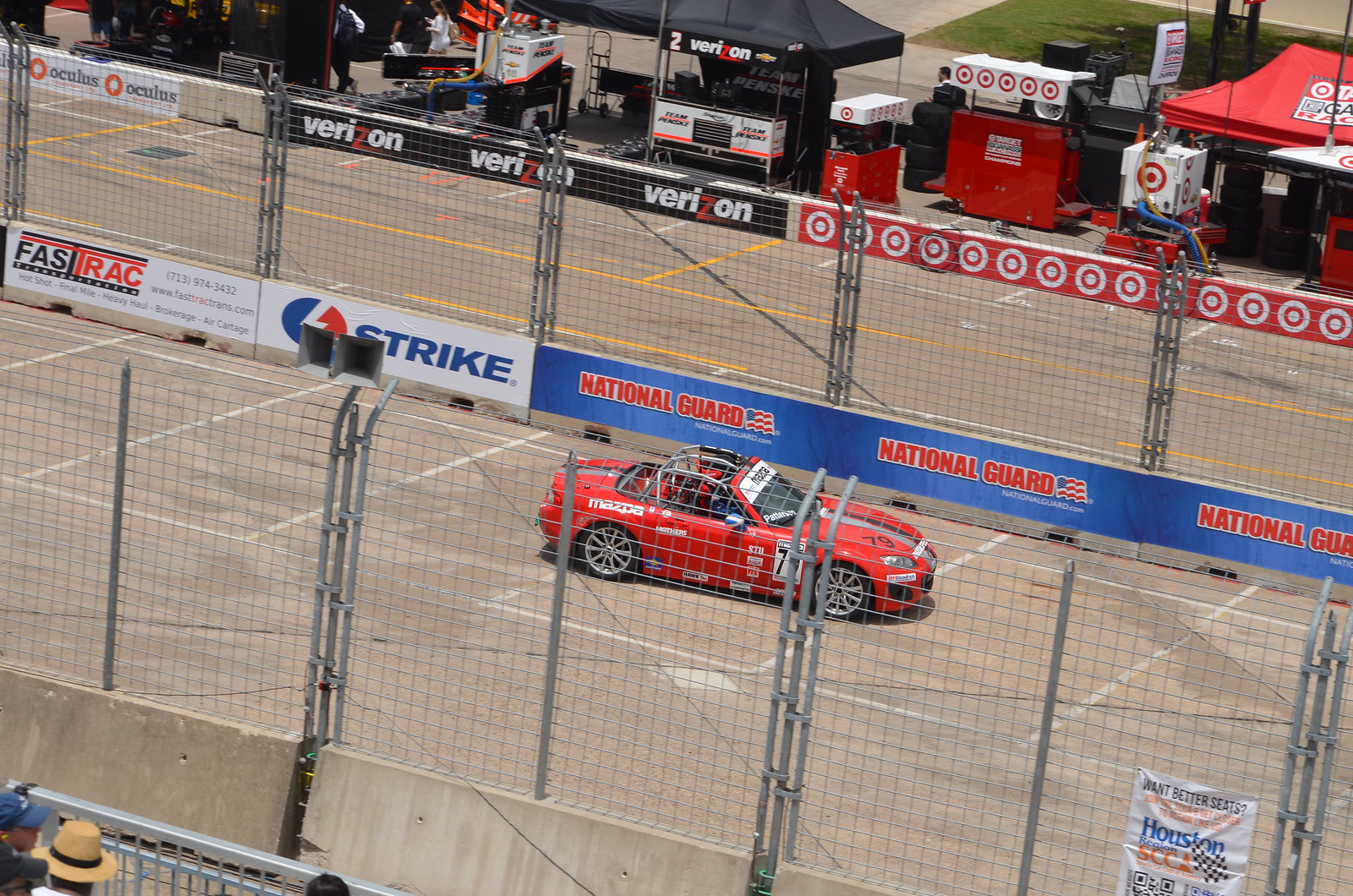This detailed photograph captures a lively scene at a racetrack, likely during a race day event. Central to the image is a striking red Mazda sports car with an open top and a robust metal roll cage, positioned prominently on the light brownish-gray cement track. The car, emblazoned with the number 79 and various stickers, appears either ready to race or just finished. Surrounding the track are sturdy metal fences, with guardrails beneath them displaying blue National Guard banners with red text, and additional banners including Strike and Fast Track on the far left.

In the lower left corner, several spectators wearing caps—one straw-colored and another blue—peek over the fence, indicating high stands from which the photo might have been taken. Beyond the track's barrier, there's a bustling pit area filled with temporary tents and awnings, showcasing multiple booths from sponsors like Oculus, Verizon (with two noticeable booths), and Target. The presence of these booths suggests the area is alive with exhibitor activities, adding to the busy atmosphere of what appears to be a daytime event, thanks to the clear lighting in the image.